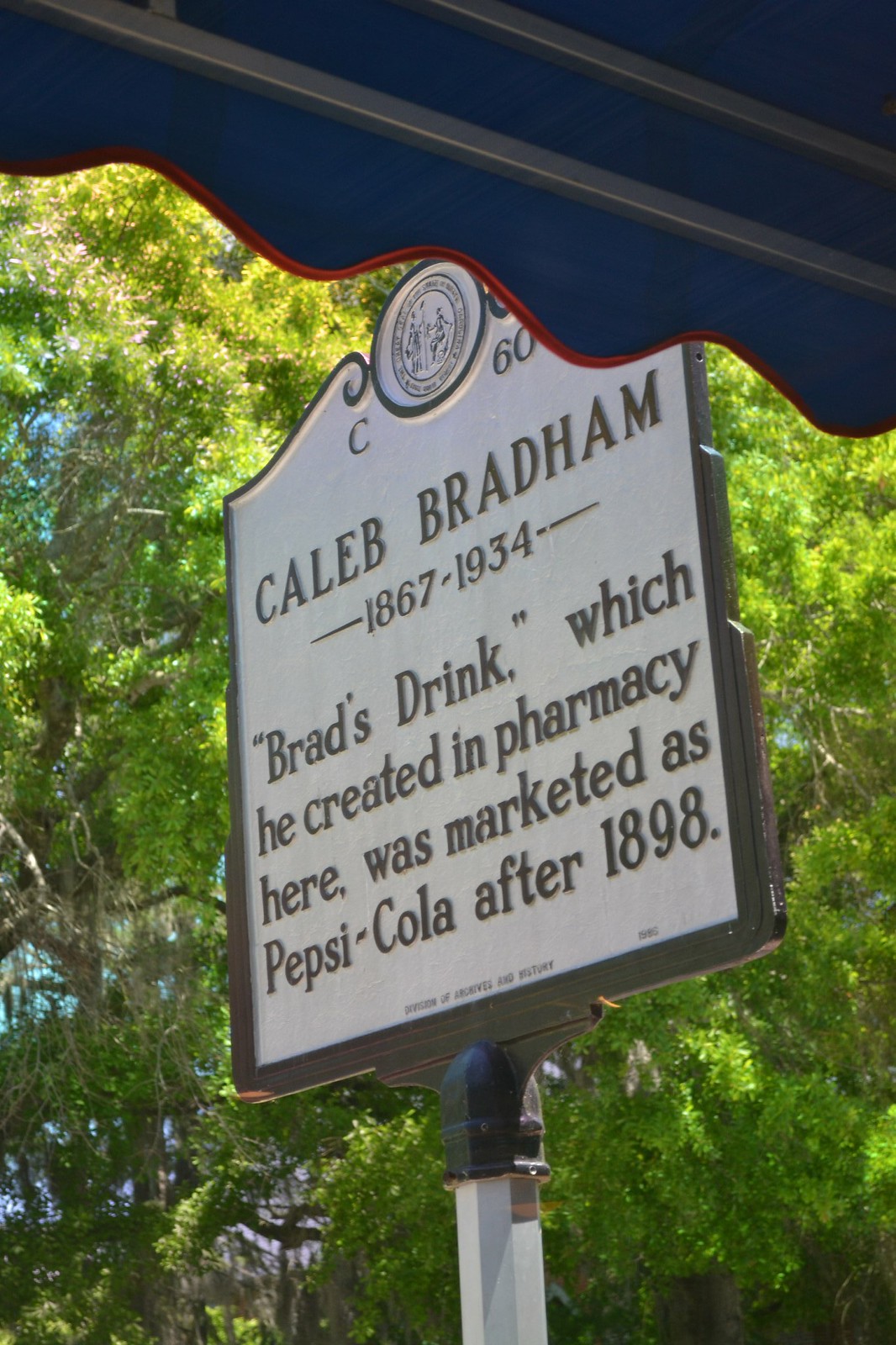The photograph depicts a historical marker in a rectangular shape, prominently featuring a bronze-colored plaque with raised black text and a black border. Topped with a circular logo, the plaque honors Caleb Bradham (1867-1934) and details how "Brad's Drink," created in his pharmacy, was rebranded as Pepsi-Cola after 1898. The plaque is mounted on a sturdy metal post. In the background, a large, leafy tree with glimpses of blue sky and a lush green canopy indicates the image was taken outdoors, likely during summer. The scene includes a blue awning with red trim that partially covers the top right corner of the plaque, hinting at the photo's perspective being from underneath this awning.